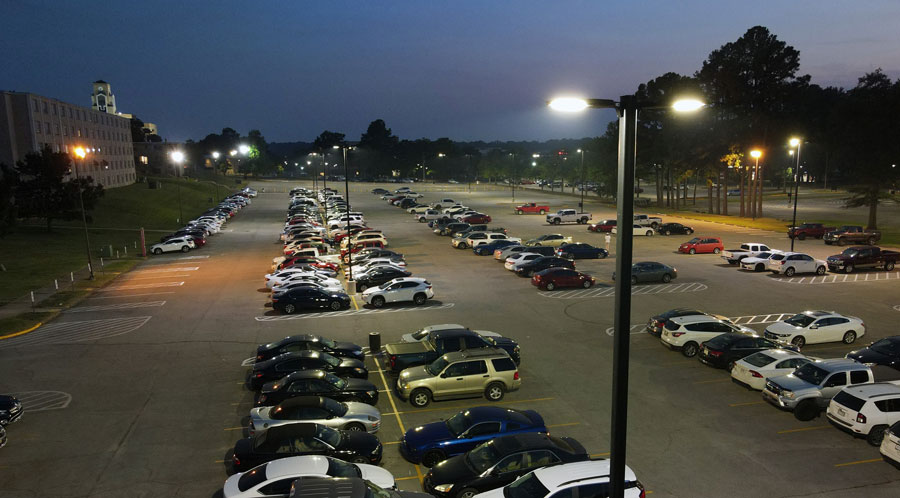This is a nighttime overhead photograph of a large, multi-row parking lot next to a complex of buildings that include a prominent five-story brown building with a bell tower and the tips of a beige building in the distance. The parking lot is well-illuminated by tall, black light poles, each with dual light fixtures that cast a yellowish to golden glow across the scene. A mix of cars, pickup trucks, and SUVs of various colors, including white, black, blue, gold, and red, fill the parking spaces, making the lot about three-quarters full with the majority of cars concentrated on the left side, a sparser collection towards the center, and even fewer on the right. On the far left of the image, a large lush green tree stands near the brown building, framed by wide grassy fields on both its left and right. Trees also line the front and side perimeters of the parking lot, and a secondary, mostly empty, parking lot is visible on the far right. The surrounding landscape, adorned with dark green trees and park-like areas, is set against a dark bluish-gray to bluish-purple sky, adding to the serene ambiance of the scene.